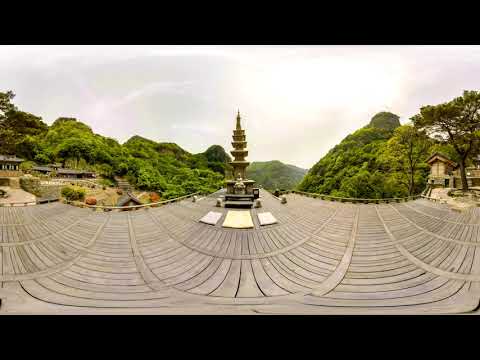This fisheye-perspective image captures a detailed outdoor scene centered around a striking temple-like monument. The central structure, resembling a layered shrine or gondola, features a large bottom that gradually narrows into a sharp point at the top, reaching towards a cloudy but slightly pink sky. The monument sits on a cement platform adorned with board or tile designs, enclosed by a fenced berm. In front of the temple, three evenly spaced squares with distinct coloration—a larger yellowish square flanked by two smaller grayish-brown squares—mark the ground. To the left, a low-standing house is partially obscured by dense, green mountain foliage. A similar house-like structure is visible to the far right. Behind the temple and across the background, tree-covered mountains rise, emphasizing the monument’s serene and picturesque setting. The scene suggests a tranquil park or memorial area, with no visible text or inscriptions.